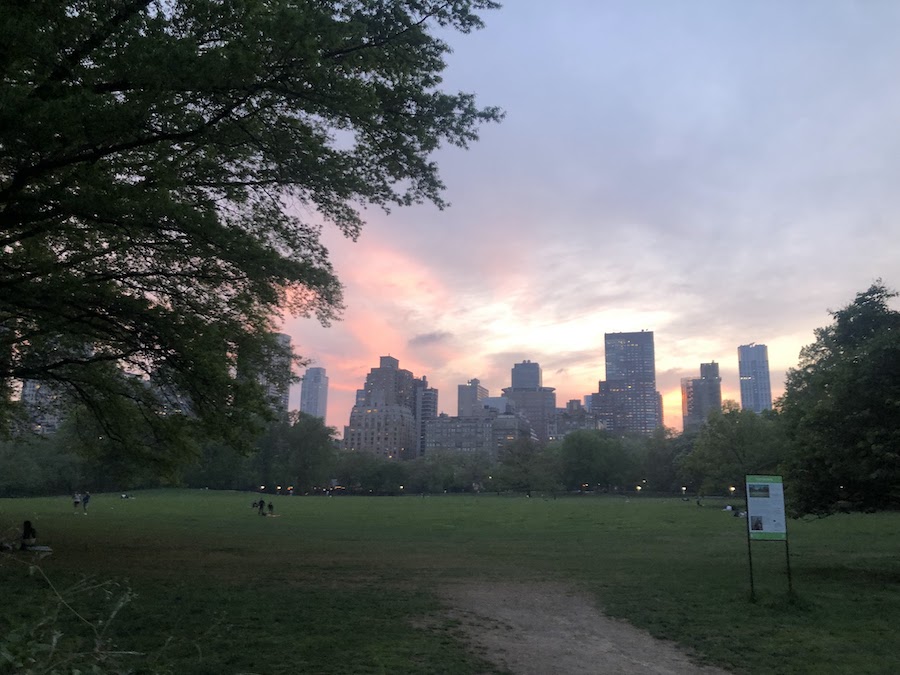This photograph captures a city park during sunset. In the foreground, a large green field is bordered by tall trees, creating a natural frame around the park. A dirt path leads into the park, ending where the green space begins. On the lower right corner, a metal sign, likely bearing park rules or information, is visible but not readable. Scattered across the park, particularly along the left side, are a few people either walking or sitting on blankets enjoying the late evening. 

A prominent, large tree in the top left corner extends its branches and partially obscures the sky. To the right side, more trees line the area, maintaining a natural border. Streetlights around the park are beginning to illuminate the scene as dusk settles in. The skyline of tall buildings stands distinctly beyond the treeline, under a sky painted in purples, oranges, and darkening blues with clouds giving the scene a somewhat gloomy feel. The overall image conveys a tranquil, almost serene ambiance as the day transitions to night.